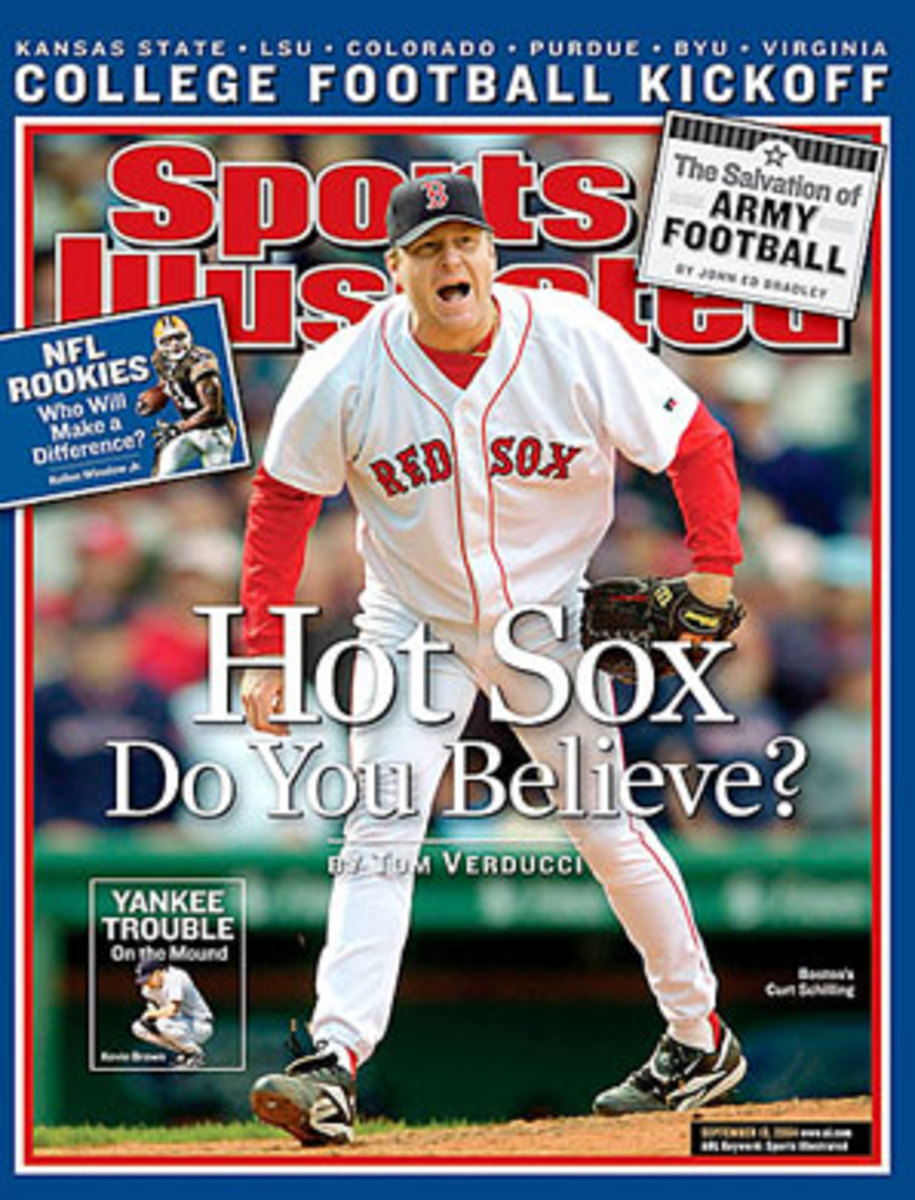The cover of Sports Illustrated features Kurt Schilling, a Boston Red Sox player, prominently in the center. The backdrop is predominantly blue, with Schilling captured mid-yell, wearing a Red Sox uniform with "Red Sox" emblazoned across his chest, a black hat with the team's logo, and a long sleeve red undershirt under his white jersey. His head and shoulders partially obscure the "Sports Illustrated" logo. The main headline splashed across Schilling's midsection reads, "Hot Sox, Do You Believe?" by Tom Verducci. At the very top, a blue header lists "Kansas State, LSU, Colorado, Purdue, BYU, Virginia," followed by "College Football Kickoff" in larger white letters. The top right features a white box with black text declaring, "The Salvation of Army Football" by John Ed Bradley. On the left side, near his arm, there is a blue box that states, "NFL Rookies Who Will Make a Difference." The bottom left corner of the cover has a transparent stamp that says, "Yankee Trouble on the Mound." Additionally, a small text box at the bottom right notes, "Baseball's Kurt Schilling." The cover design includes a tripartite frame with blue, white, and red layers.